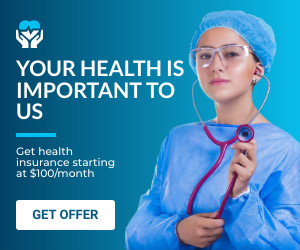The advertisement showcases a healthcare or health insurance program, prominently featuring a square image with a blue background. On the right side, there is a professional, female nurse adorned in a blue cap and a matching long-sleeve gown. She has a stethoscope placed around her neck, holding its diaphragm in her left hand. The nurse, with light tan skin, conveys a sense of care and professionalism.

To her left, the ad features a clear and compelling message in white text: "Your health is important to us." Beneath this, smaller white text states, "Get health insurance starting at $100 a month." At the bottom left corner, there is a clickable white rectangle button with the text "Get Offer" in blue, inviting viewers to take action.

At the top left, a company logo is displayed: a pair of white hands cradling a heart. The heart is uniquely designed with its top half in blue and the bottom half in white, separated by a line representing a heartbeat monitor’s waveform. This logo symbolizes care and medical assurance, enhancing the trustworthiness of the advertisement.